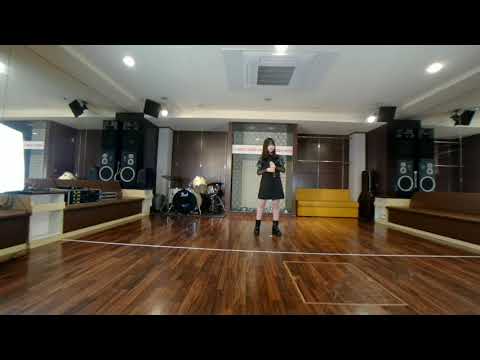A low-resolution photorealistic image reveals the interior of a dance studio or rehearsal room. The room features a glossy, brown-patterned wooden floor with a white line crossing it in front of the central figure. The side walls are mirrored and adorned with black speakers, while the back wall is brown paneled, interrupted by a gray segment with a white band running across the top. In the room's center, slightly right of the image's center, stands a girl with long dark hair, dressed in a black dress and matching boots, holding an indeterminate object. To her left is a black and white drum set, positioned on the back left. In the back right corner, a square yellow couch is situated. The photograph is wide and rectangular with black bars cropping the image at the top and bottom. The ceiling of the room is white, contributing to the overall bright atmosphere of the space.